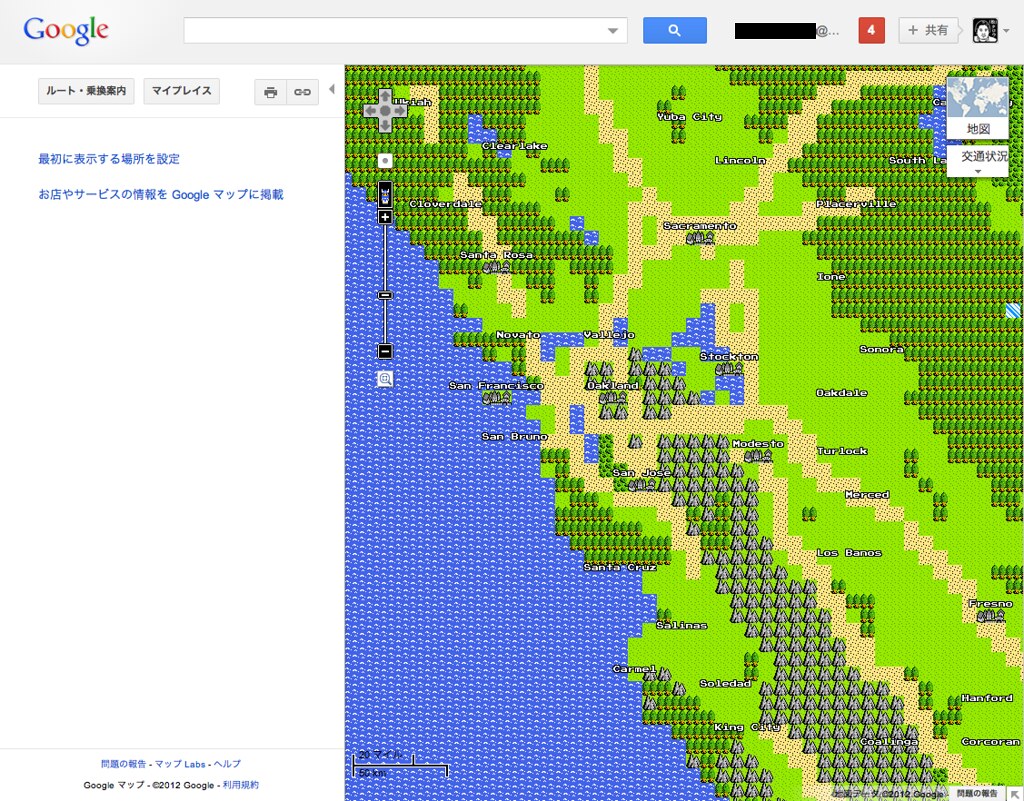This image depicts a computer screen displaying a Google search bar at the top, with the iconic multi-colored "Google" logo to the left. Below the search bar, there appears to be a directions map that resembles the coast of California. The map is quite pixelated, with blue water visible on the left side and green land to the right, featuring several blue lakes. There are navigation arrows for scrolling vertically. In one corner, there is a small globe icon. The text on the screen is written in a foreign language, likely an East Asian script, indicating that the map might be from an oriental country.